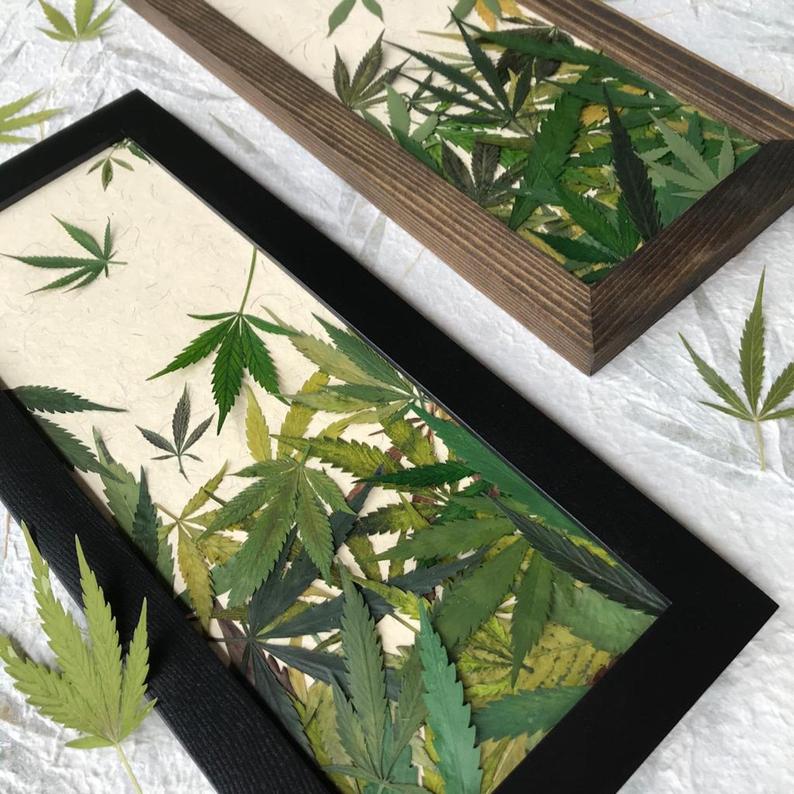The photograph showcases two vertical rectangular picture frames, artistically filled with vibrant cannabis leaves of varying green shades and forms. These frames rest askew on a white fabric tablecloth adorned with matching leaf patterns. The left frame is sleek black, while the right frame boasts a rich dark brown wood grain. Inside each frame, the cannabis leaves, distinctively characterized by their multiple stems and spiked edges, appear as if cascading into a gentle pile, with denser clusters at the bottom gradually thinning towards the top. Complementing the framed designs, additional cannabis leaves are scattered around the frames and leaning against them, all set against a tannish-white background marked with subtle black lines.